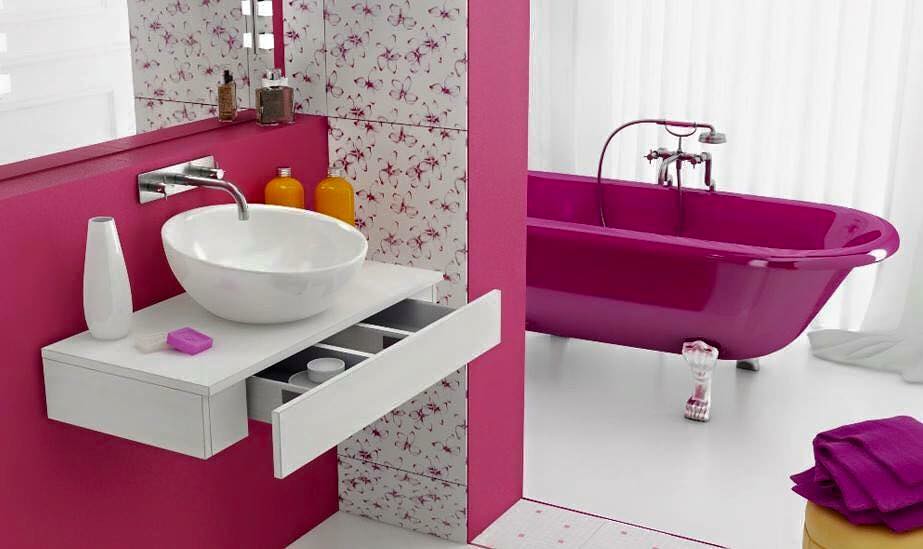The image is a meticulously staged and aesthetically pleasing interior shot of a luxurious bathroom, designed to evoke a sense of elegance and charm as if intended for a magazine spread or an artistic display. The photograph captures a wide landscape view in vibrant color, focusing on both foreground and background elements.

In the foreground, there is a sleek, wall-mounted vanity featuring a stylish sink and an immaculate mirror, all exuding modern sophistication. To the right of this vanity, a narrow, diagonal partition wall extends outward, approximately one foot long and half a foot deep. This wall projects at an angle, with its front edge aligned towards a four o'clock position, effectively creating a visual separation from the bathtub area behind it.

Dominating the background is a standout piece: a pink claw-footed bathtub with gleaming silver feet that reflect light. The positioning of the bathtub runs parallel to the diagonal partition wall but is partially obscured by it, with the tub extending horizontally behind the wall. The far end of the tub features a classic tap setup, including a left and right separate mixer with cross-shaped handles, reminiscent of clock hands at the 12, 3, 6, and 9 positions. Adjacent to the taps is a handheld shower head, elegantly curved downward into the bath and mounted on a holder shaped like an inverted rainbow, with the shower head pointing right.

Further enhancing the room's cohesive color theme, the foreground under that vanity shows an open drawer, drawing attention to practical yet sophisticated storage. Pink accents are prominent throughout, including a neatly placed pink bar of soap and a plush pink towel on the right side of the foreground. These elements reinforce the luxurious, coordinated atmosphere of the pink-themed bathroom, making it a quintessential example of refined interior design.